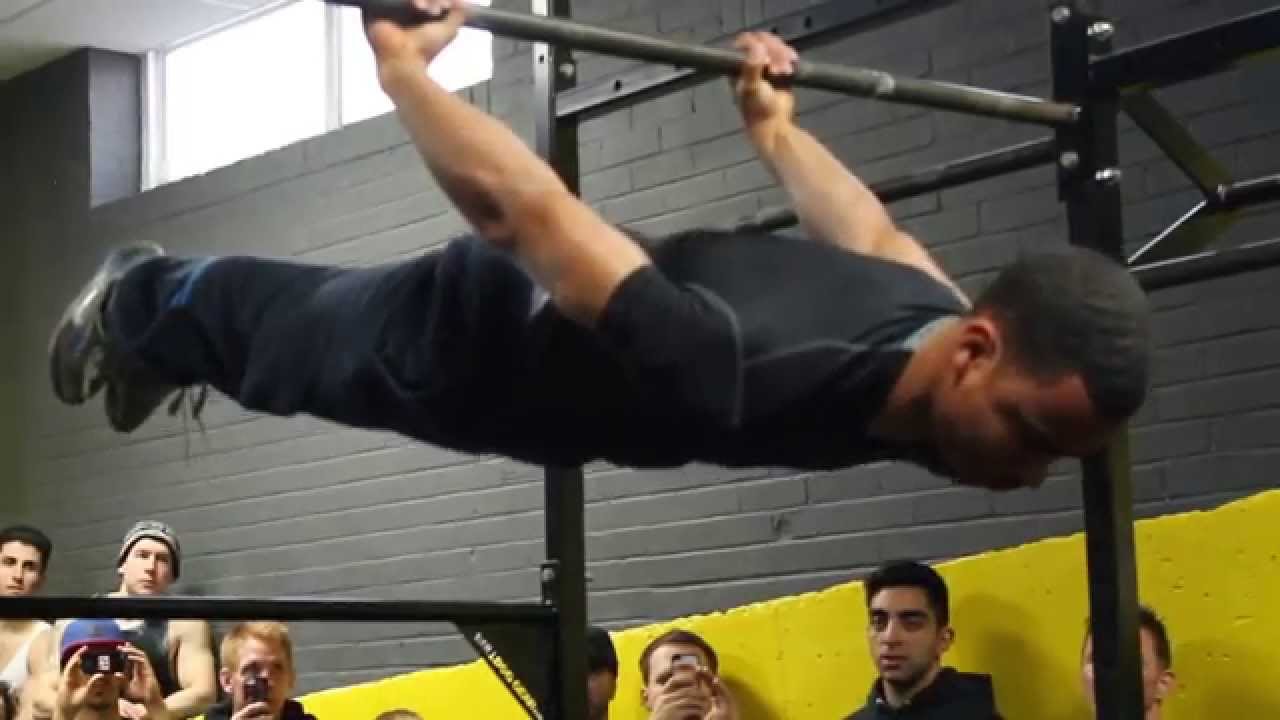In the image, a male gymnast is performing an impressive horizontal hold, with his back facing a metal exercise bar. Dressed entirely in black, including a black shirt, black joggers, and black tennis shoes, he is suspended mid-air in a prone position, with his body perfectly straight as if planking. His arms are fully extended behind him, gripping the bar firmly above and behind his back. In the background, there is a gray brick wall with its lower section painted yellow, and a long window at the upper left corner of the wall allows sunlight to filter through. Seven onlookers are present, with three of them actively taking pictures or recording the performance using their camera phones. The setting appears to be a gym, where the gymnast is possibly demonstrating techniques to a group of students.